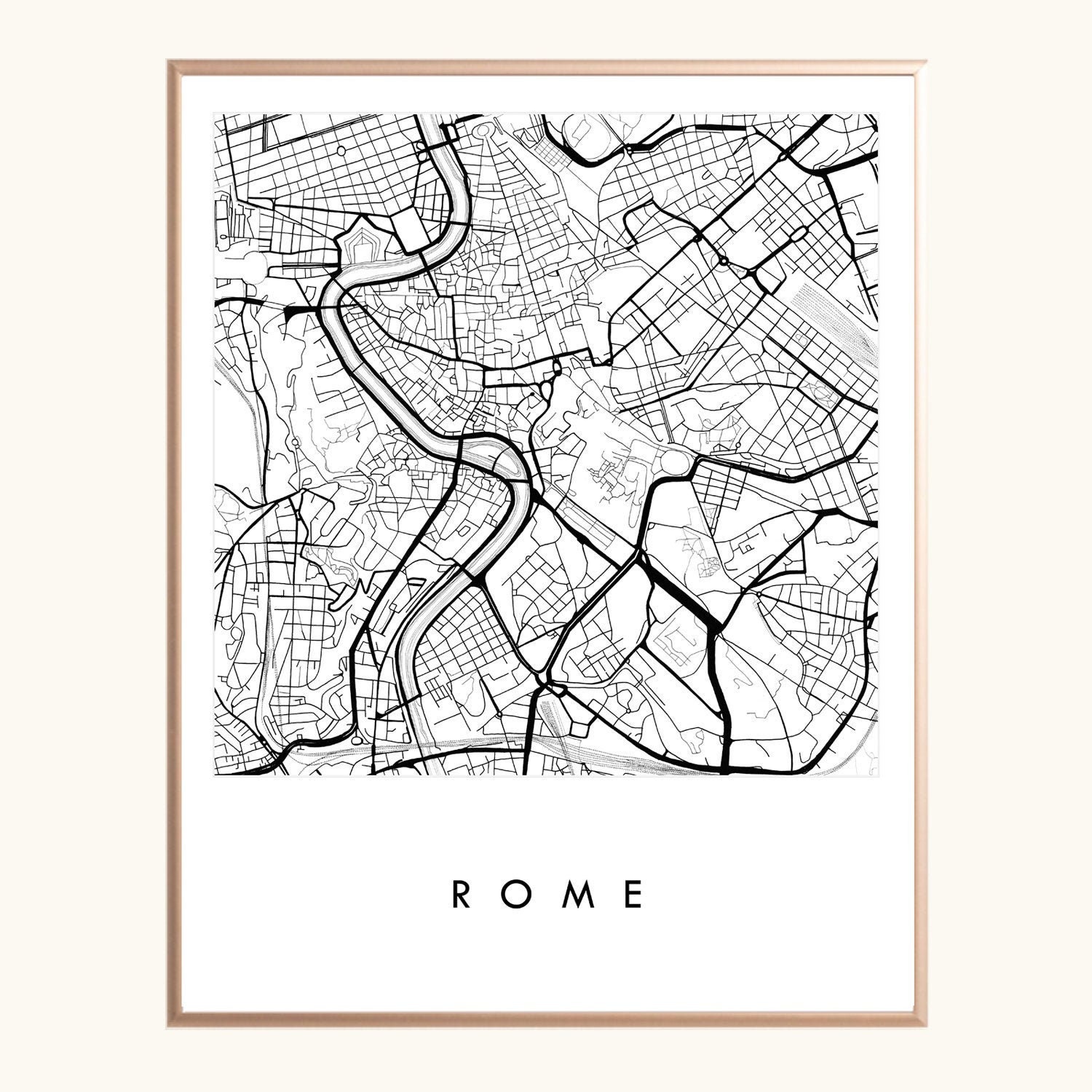This vertically rectangular image features a detailed black and white map of Rome. The map itself, void of any labels, showcases an intricate network of streets and a river flowing through the city. It is framed by a simple, thin wooden frame, with an off-white border surrounding the entire composition, which is thicker on the sides than on the top and bottom. The word "ROME" is prominently displayed in all caps at the bottom center of the image in black text. The overall aesthetic is minimalist and monochromatic, combining clean lines and contrasting shades to create a visually striking representation of the city's layout.